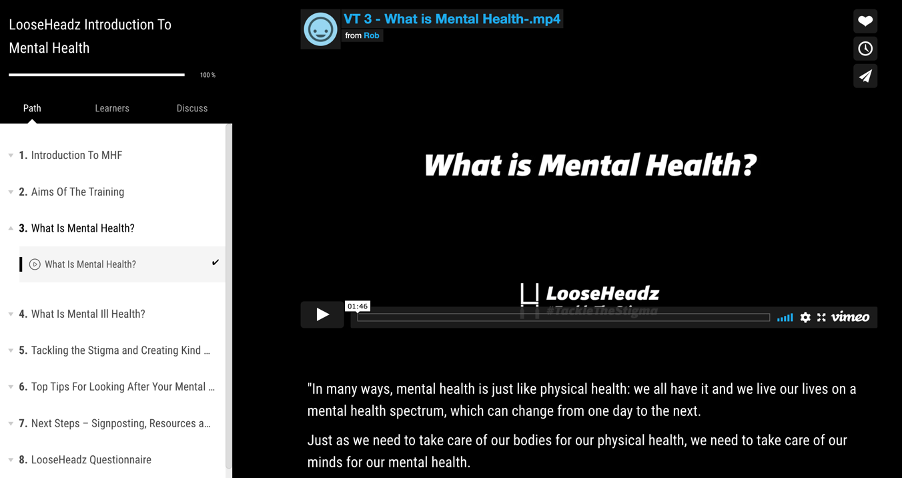The image features a predominantly black background with white text at the top left that reads "Loose Heads Introduction to Mental Health," where "Loose Heads" is distinctly spelled "L-O-O-S-E-H-E-A-D-Z." At the top center in blue text, it says "VT3-WhatIsMentalHealth-.mp4," accompanied by a light blue circle containing a simple smiley face illustration. 

Just below the middle, in italic white text, the caption reads "What Is Mental Health?" This is followed by a video from Vimeo, which prominently features the logo "Loose Heads." At the bottom, a paragraph in white text articulates the message: 

"In many ways, mental health is just like physical health. We all have it, and we live our lives on a mental health spectrum, which can change from one day to the next. Just as we need to take care of our bodies for our physical health, we need to take care of our minds for our mental health."